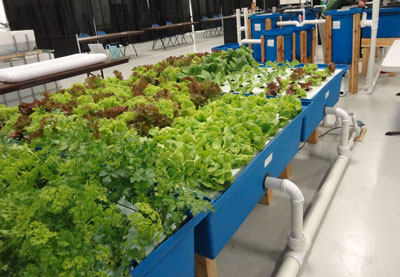This indoor photographic image captures an intricately designed aquaponics garden. Dominating the scene are a series of large blue rectangular containers arranged diagonally from the bottom left to the center-right of the image. These containers are connected by white water pipes, originating from a main pipe that runs along the white floor in the bottom right corner. The pipes extend upwards and curve into each container, delivering water essential for the flourishing plants within.

The plants are predominantly green, though some feature purple or brown hues. In the middle container, there are some reddish or brownish plants adding contrast to the lush greenery. The garden's layout includes blue containers dotted throughout, with each container showcasing a variety of plants at different growth stages. In the background, a network of white rails or pipes, brown posts, and additional blue containers can be seen, creating a structured environment for optimal plant growth.

To the left and top-left of the image, there are wooden stands and a table draped with a white cloth, adding a touch of homeliness to the otherwise industrial setup. The upper right corner reveals smaller green and brown plants, while adjacent to them in the far background, some larger plant varieties are visible. The backdrop also features an array of blue and white cylindrical structures and potential storage spots, adding depth and additional context to this vibrant indoor garden scene.